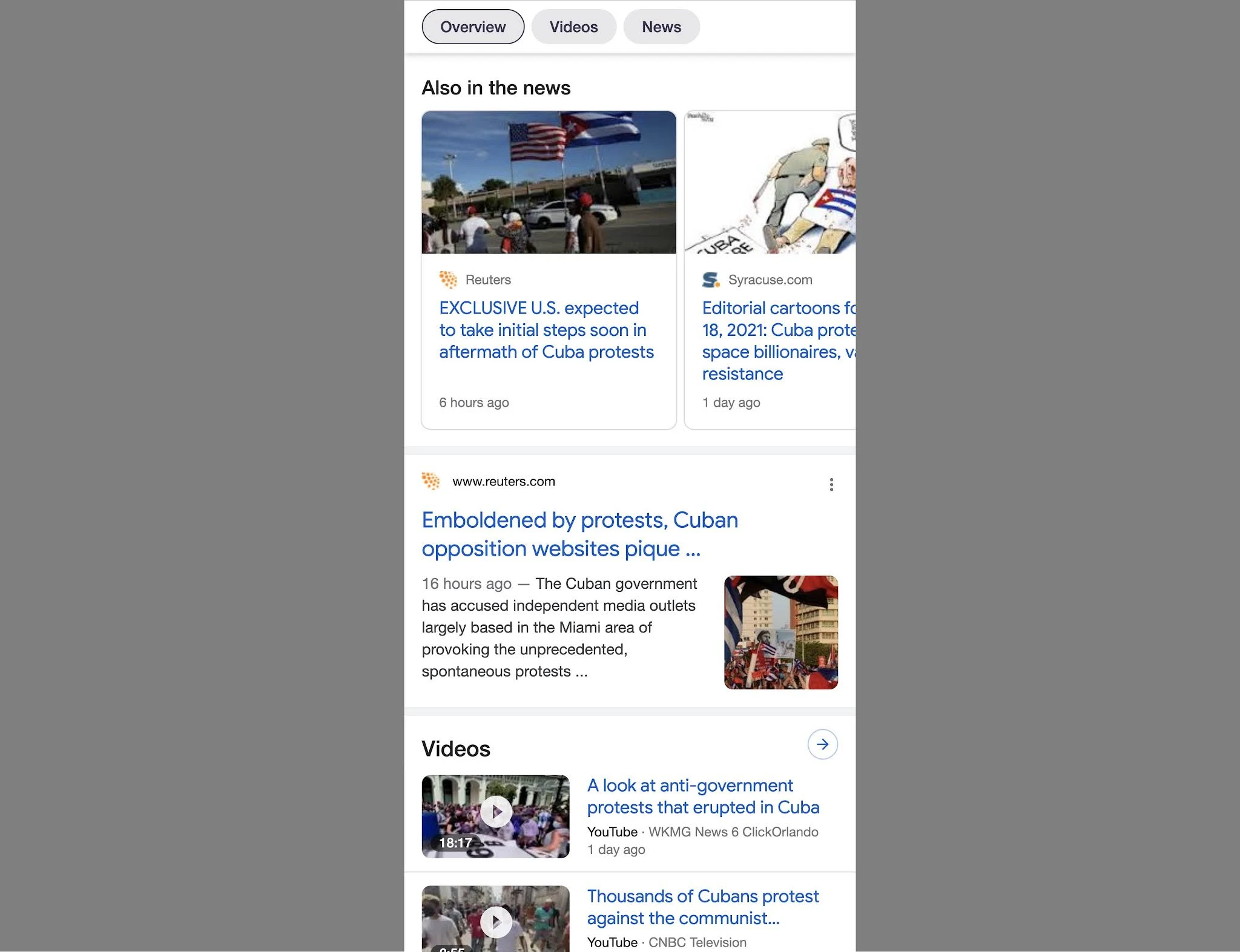**Detailed Descriptive Caption:**

This image is a vertical screenshot that appears to have been captured on a smartphone. On each side of the screenshot are vertical dark gray bars, indicating that the image itself has been framed within these margins. At the top of the screenshot, there are small horizontal navigation bubbles labeled "Overview," "Videos," and "News" in black text, indicating different sections of content.

In the "News" section, several articles are displayed. The first article, from Reuters, has a headline that reads: "Exclusive: U.S. expected to take initial steps soon in aftermath of Cuba protests," with a timestamp indicating it was posted six hours ago. The next entry appears to be an editorial cartoon from Syracuse.com, but most of the text and illustration are cut off and the date reads "4/18/21."

Following that, another Reuters article is titled, "Emboldened by protests, Cuban opposition websites peak." This article, posted 16 hours ago, includes details about the Cuban government's accusations against independent media outlets based mostly in the Miami area, alleging that they have provoked the unprecedented, spontaneous protests.

Beneath the news articles, the screenshot transitions to the "Videos" section, highlighted with a black heading. There are two videos shown, but their thumbnails are obscured and only the white play button is visible. The text accompanying the videos says: "A look at anti-government protests that erupted in Cuba," and "Thousands of Cubans protest against the communist."